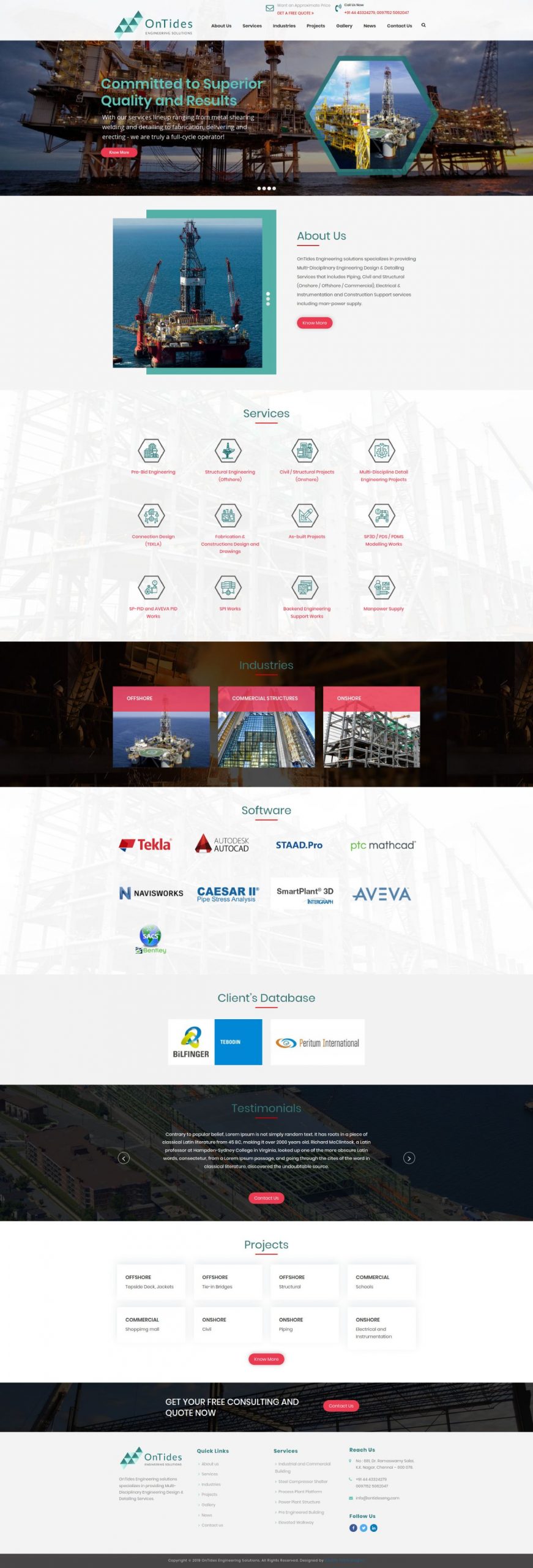This detailed screenshot of a website showcases different oil rigs. At the top, a grey navigation bar spans the entire width of the page. On the left side of this bar, there is a logo for "On Tides," depicted in green and composed of six triangles arranged to form a cohesive shape. 

The navigation menu includes seven grey buttons serving as options for navigating the website. Below this, a large banner image features an oil rig, portraying the site's primary subject matter. Overlaid on the right side of this banner is a hexagon-shaped picture, adding a layer of visual interest. On the left side of the banner, a green text reads, "Committed to Superior Quality and Results," highlighting the company's dedication to excellence.